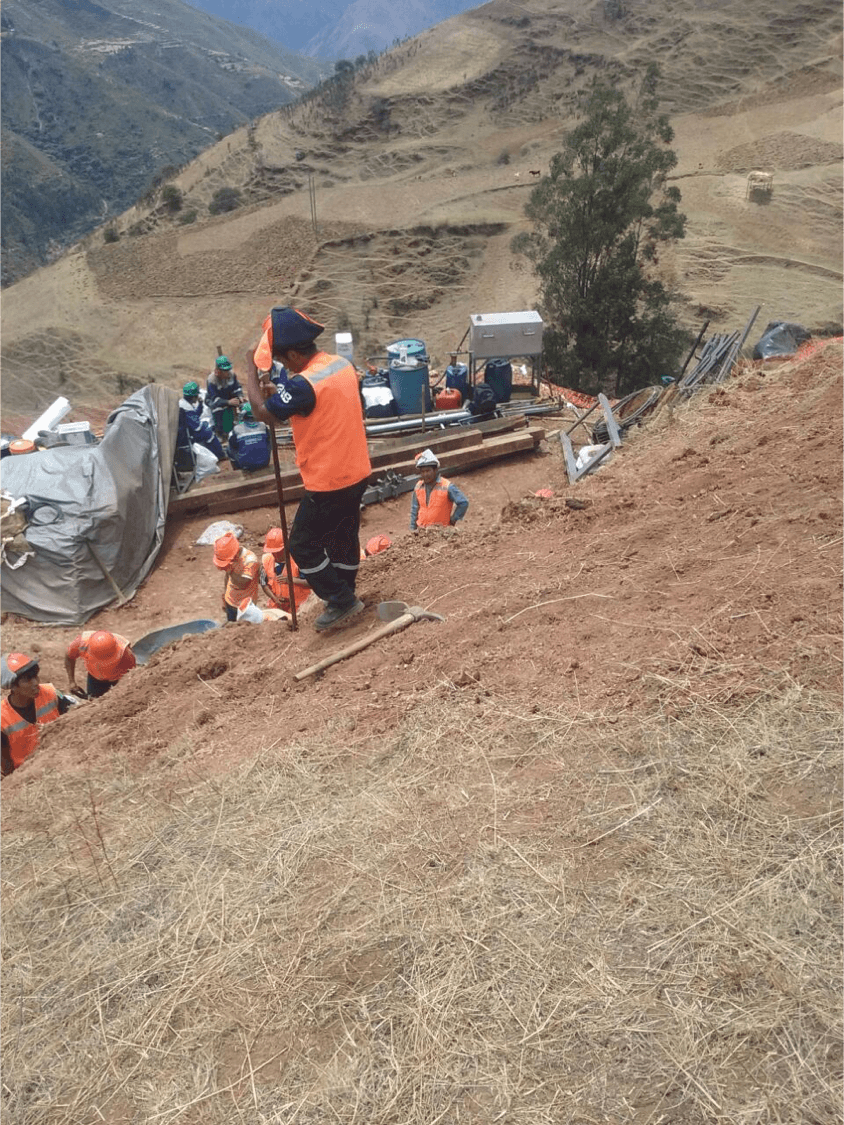The image showcases a construction site on a hillside in a mountainous region, featuring several construction workers. The workers, dressed in orange jackets and helmets, are dispersed across the sloped terrain. Dominating the scene is a worker standing centrally near the top of the hill, holding a crowbar with a pickaxe lying behind him. Behind this central figure are barrels and beams, with another group of workers, some wearing blue outfits, observed sitting and conversing. To the top right of the image, a tree stands prominently, while the background reveals a distant mountainous landscape under broad daylight. A tent-like structure or tarp is visible to the far left, contributing to the scene’s industrious ambiance.